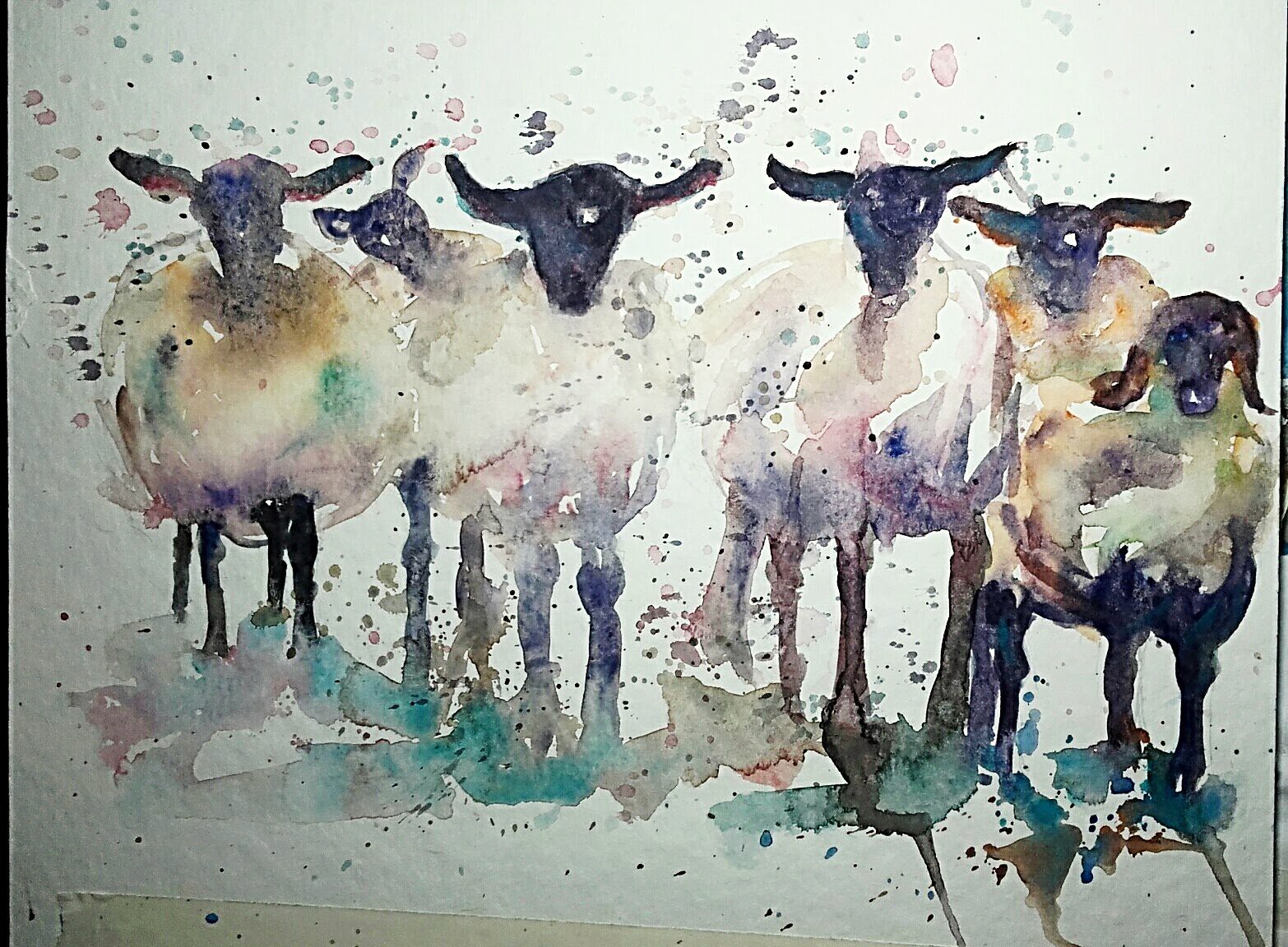This image is a photograph of a watercolor painting depicting seven fluffy, black-faced sheep. Each sheep stands in a row, facing the viewer, and they are rendered with artistic splashes of color including shades of grey, blue, purple, and green. The texture of their wool, achieved through the artist's use of browns, creams, pinks, and mauves, conveys a surprisingly convincing white appearance despite the atypical hues. The black ears and legs add contrast, while beneath their feet, the watercolor transitions into shades of blue and brown, suggesting shadow and ground. A light splatter of various colors, possibly applied with a toothbrush, extends above the sheep’s heads, adding a whimsical touch to the composition. A small piece of masking tape is visible at the bottom, hinting at the artwork's physical nature as a photograph of a watercolor painting. The background, primarily white, carries a slight green tint due to lighting. There is no text in the image.